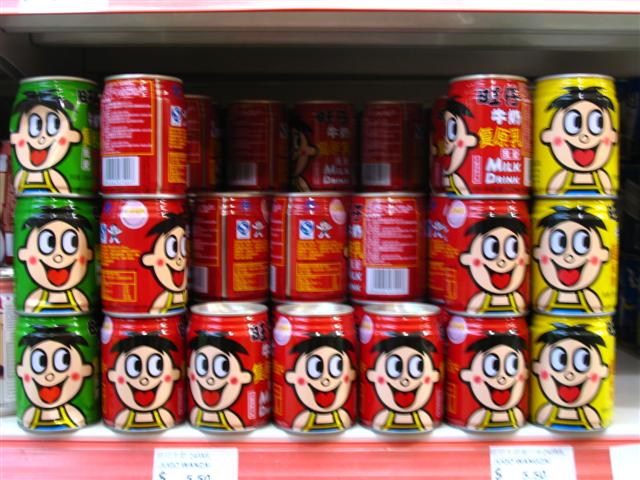This image depicts a grocery store shelf with a distinct arrangement of colorful beverage cans, each featuring a playful cartoon character. The shelf front is red with white price labels, partly blurry but suggesting foreign text, likely Chinese or Japanese. The cans are organized into five visible columns and three rows, making a total of fifteen rows, although it appears that approximately nine cans are missing from the central columns. The cans themselves feature a character with wide-open, big white eyes looking to the right, a heart-shaped tongue sticking out, and a small patch of black hair resembling a toupee. The character wears a yellow outfit, possibly a tank top or apron. The cans on the leftmost column are green, while those in the rightmost column are yellow. The three central columns are red, some displaying the text "milk drink" alongside Asian characters. This meticulous arrangement and the colorful aesthetic make the display eye-catching and unique.